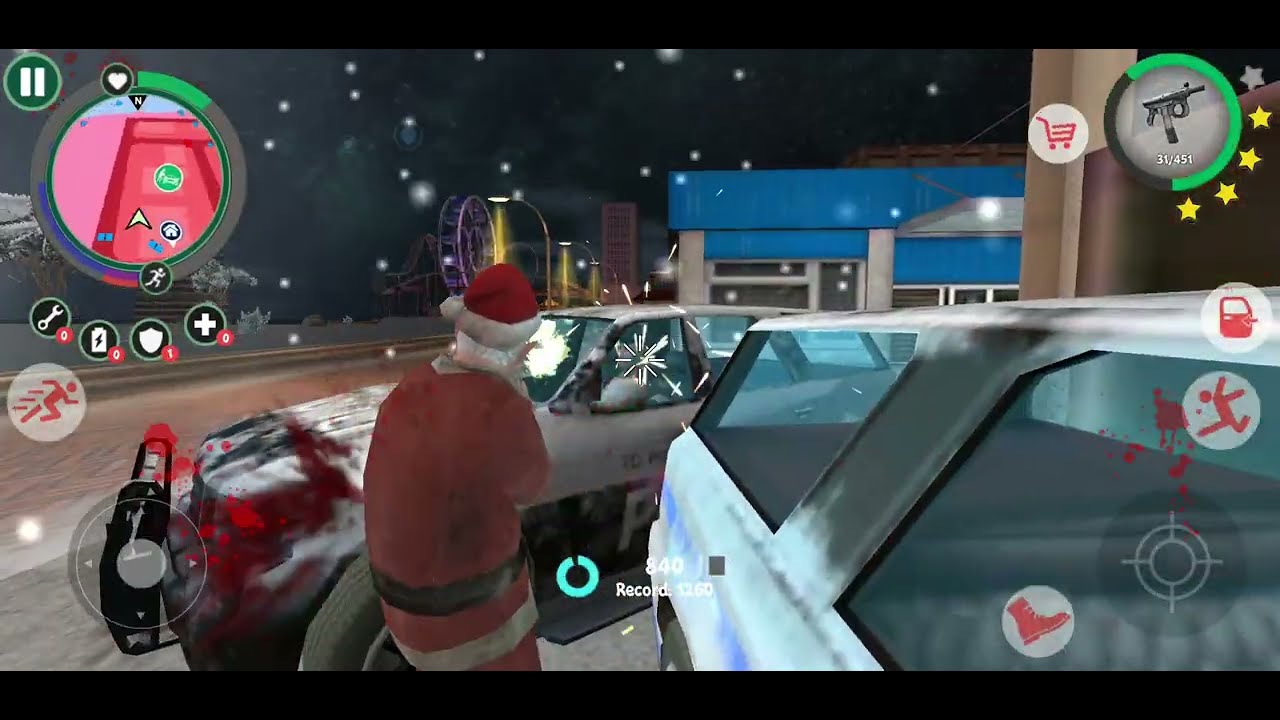The image is a detailed screenshot from a colorful, cartoon-like mobile shooting game set in a vibrant, night-time cityscape. The character, dressed as Santa Claus, is centrally positioned and seen from the back, holding a gun and shooting at a car, which is splattered with red blood. There are two vehicles strategically used as barriers for cover. 

In the upper left corner of the screen, a minimap displays the character's location with a triangle. Beside it, a heart icon indicates remaining health, accompanied by a pause button and four utility icons including a wrench, a battery, a shield, and a plus sign for various game functions. 

The upper right-hand corner features a weapon icon, likely a small submachine gun, with a green bar to show remaining ammunition. The bottom right-hand corner of the screen includes shortcut icons for an aiming indicator, a boot for movement, a jump icon, and a door icon possibly for interacting with the environment. The bottom left-hand corner has an arrow indicator for movement and a running icon above it.

The game's rich environment features an electric blue building, a Ferris wheel, and a cityscape background, creating an engaging and immersive scenario for the player.